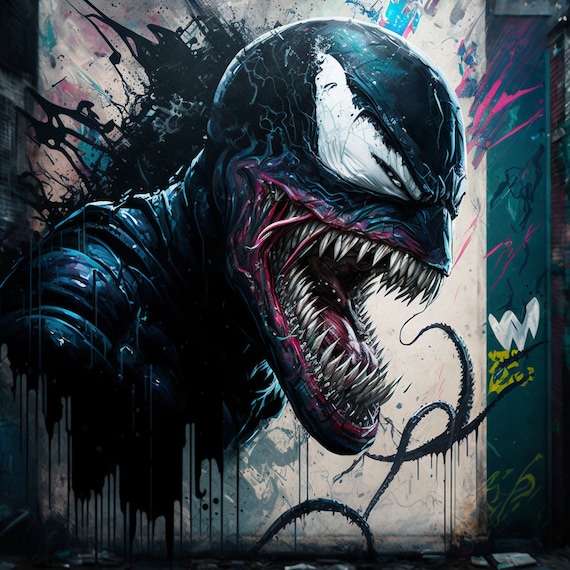The image depicts a detailed painting or colored drawing of the Marvel character Venom, known for its dark and sinister appearance. The central focus is on Venom's side profile, featuring a black head with large, triangular white eyes that have black slits. Venom's mouth is open wide, revealing numerous sharp white fangs, a pink tongue, and some blue tones around the lower jaw. Tentacle-like tendrils are visible near the mouth, adding to the creature's menacing look.

The background consists of a gradient of gray hues with splashes of blue and red paint, giving it an abstract feel. There are also notable paint drips, especially around the shoulders and neck, suggesting an expressive, fluid art style. Behind Venom, the background transitions from a lighter white area to a darker greenish hue, with white and yellow squiggles adding dynamic texture. A prominent 'W' is painted near Venom's mouth, alongside other abstract markings that accentuate the chaotic background. The bottom part of Venom's figure fades into more paint drips, blending into the background and enhancing the overall composition of the artwork.